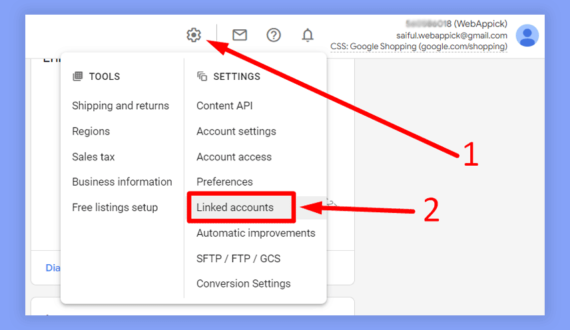The image depicts an admin page for Google Shopping, specifically an instructional or walkthrough guide. In the upper right corner, there's a blurred menu, with the name "WebEpic" followed by "APICK" and the email "Saiful.WebEpic@gmail.com" within brackets, adjacent to a generic profile icon. The label reads "CSS, Google Shopping (google.com/shopping)." 

On the top left, there's a settings gear icon highlighted, with a long red arrow labeled "1" pointing at it. Next to the gear icon, there's an envelope, a question mark, and a bell icon.

The main panel contains various tool options including "Shipping Returns," "Region," "Sales Tax," "Business Info," and "Free Listing Setup." To the right, under "Settings," there are options such as "Content API," "Account Settings," "Account Access," "Preferences," "Linked Accounts," "Automatic Improvements," "SFTP," "FTP," "GCS," and "Conversion Settings." A large red rectangle highlights "Linked Accounts," accompanied by another red arrow labeled "2" from the right.

Overall, this instructional panel appears to guide users through specific settings or features of the Google Shopping admin interface, though its exact purpose remains unclear.